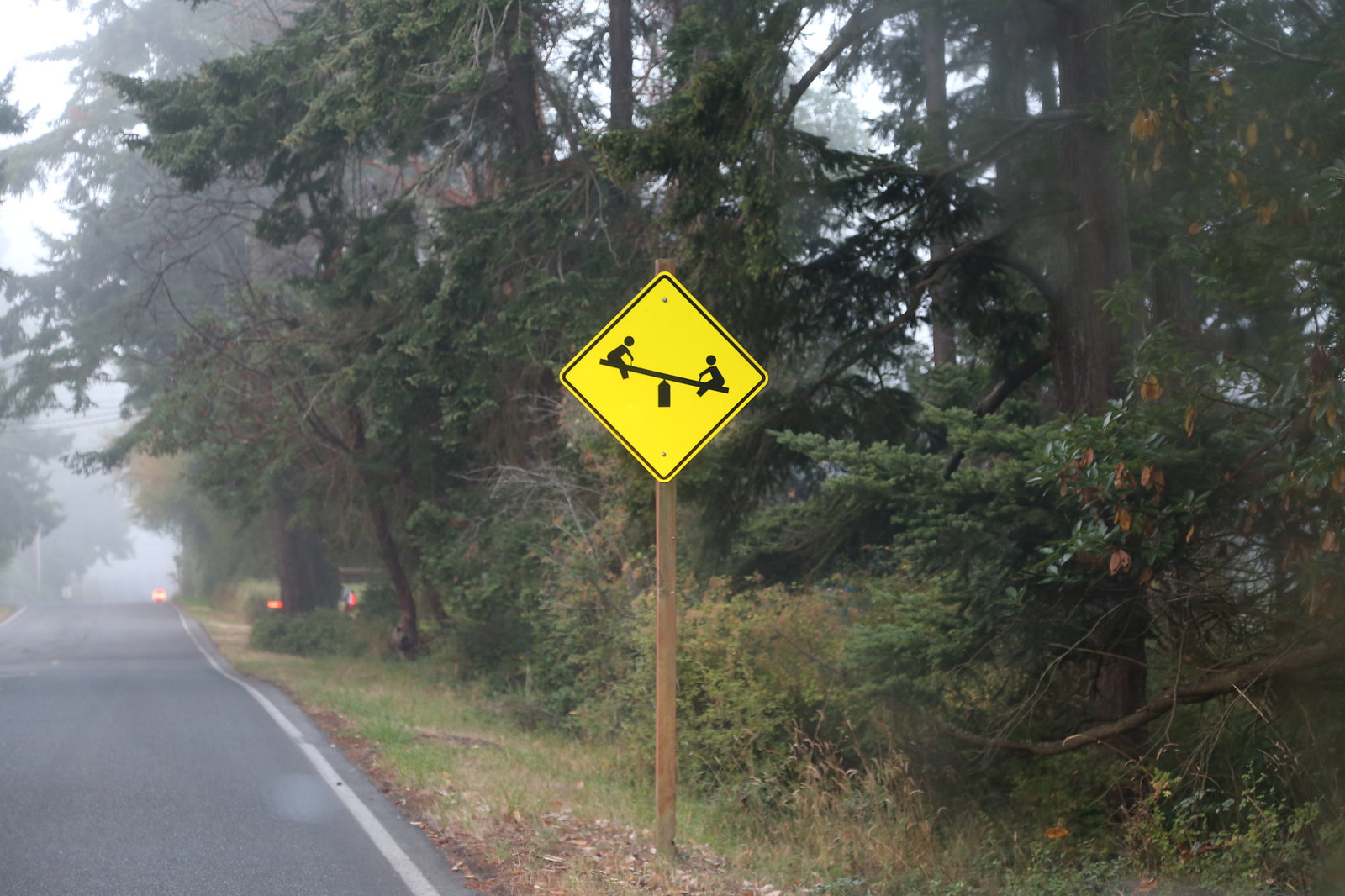This photograph captures a yellow, diamond-shaped road sign mounted on a wooden pole, positioned on the right side of a foggy, forested road. The sign features a black silhouette of a teeter-totter with two children at either end, indicating a nearby playground. Behind the sign, the dense forest comprises a mix of towering pine trees and low bushes, shrouded in mist. To the left, the asphalt road with crisp white lane markings stretches into the distance, where faint headlights are visible through the thick fog, adding to the photo's eerie and atmospheric feel.